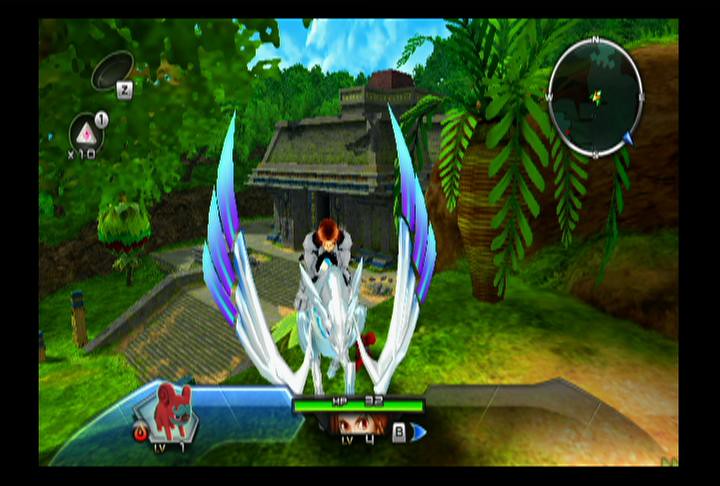The image appears to be a screenshot taken from a digital device, possibly a phone, tablet, or computer monitor, displaying a scene from a video game. In the foreground, a majestic bird-like creature, possibly a humanoid bird-person or a dragon, is prominently featured. A woman is depicted seated atop this dragon-like entity, suggesting she is either riding or in control of it. Below the creature, partially obscured by a green band, another character can be seen peeking out, potentially seeking or observing the dragon and its rider.

In the upper right corner of the screen, a compass is visible, indicating directions with "N" for north, "E" for east, "S" for south, and "W" for west. The compass needle is pointing towards the northeast, hinting at the direction the characters might be headed. The setting appears to be a dense, lush jungle, suggesting a location reminiscent of South American landscapes, potentially with Aztec or Asian architectural influences. Additionally, a red-marked cat-like creature or unit is visible at the bottom of the screen, possibly indicating another character or entity within the game.